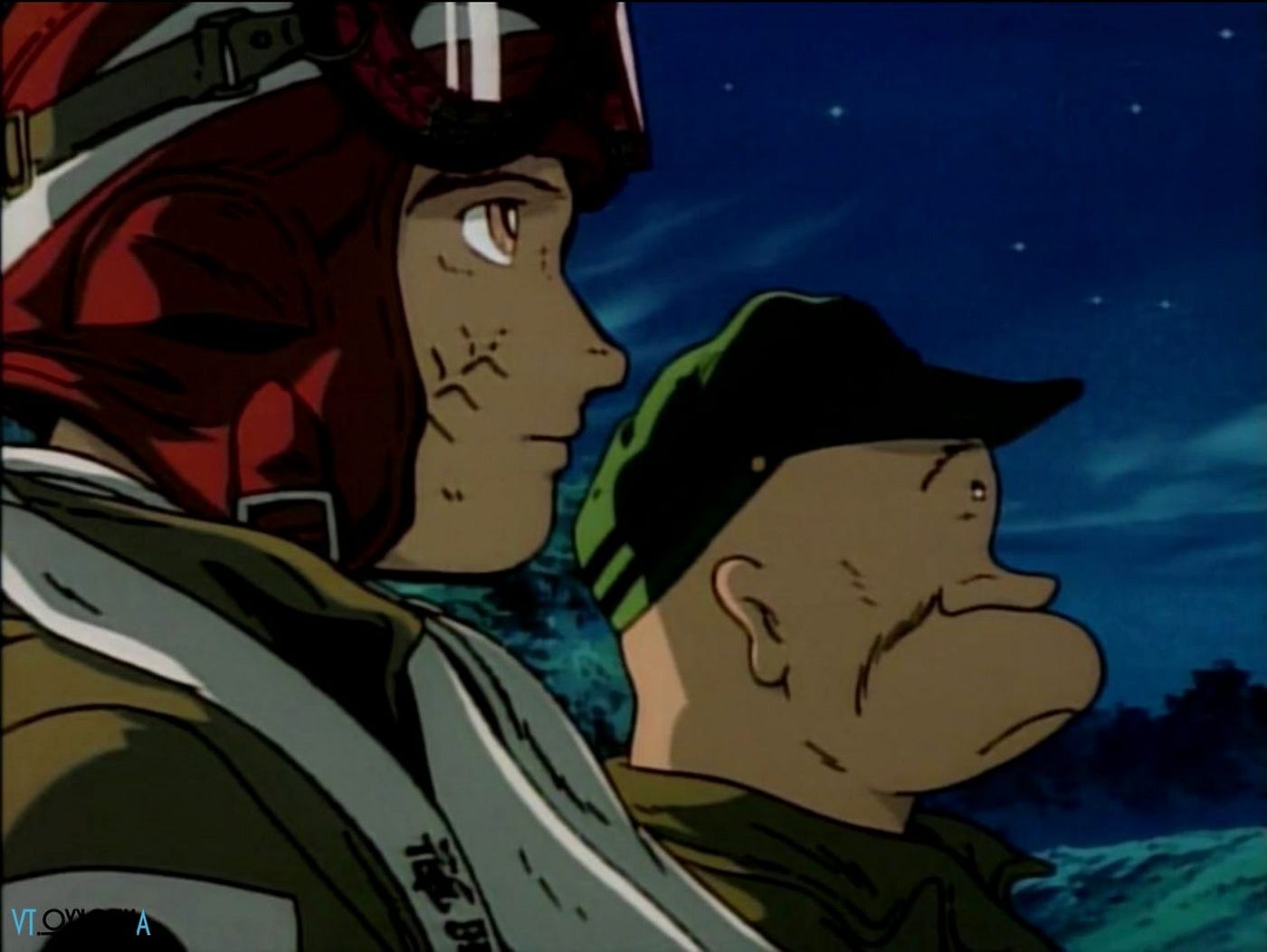This detailed cartoon image features the iconic Speed Racer prominently on the left, taking up about half of the visual space. Speed Racer, identifiable by his red helmet with a white stripe and racing goggles resting on top, is distinguished by his white scarf and visible half profile looking to the right, revealing his brown eyes and a small scar on his cheek. Adjacent to Speed Racer is an older man with a pronounced, protruding chin, wearing a green cap and a matching green collared long-sleeved shirt. Both characters are facing the same direction, towards the right. The backdrop is a medium dark blue sky dotted with small stars, with silhouettes of trees visible at the bottom of the image, lending a night-time ambiance to the scene. The perspective slightly distorts the relative heights of the characters, making Speed Racer appear taller.